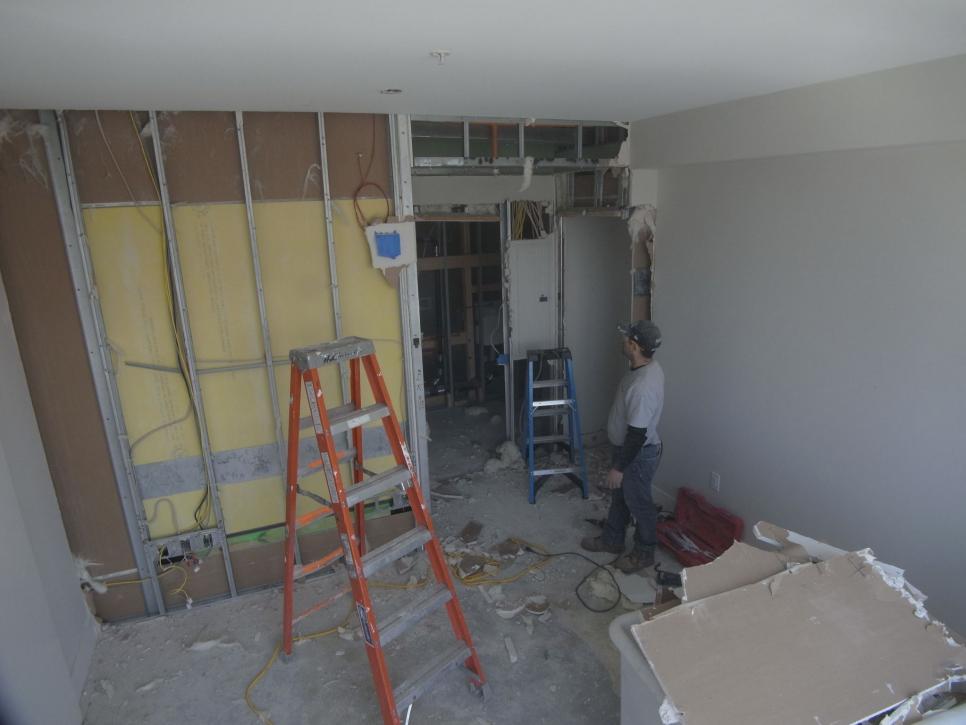The image depicts a tradesperson in the midst of a major renovation project, dressed in blue pants, grey boots, a grey short-sleeve top over a long black sleeve shirt, and a grey cap. To his left stands an orange and grey ladder, while a shorter, blue and grey ladder is positioned in front of him. The setting appears to be a spacious room with a grey concrete floor, partially torn up. Behind the tradesperson are a clear plastic bucket filled with debris, including broken drywall pieces, and an open red toolbox, with a black cord sprawled across the floor. 

To the right, there's a hallway where the metal framing of the ceiling is visible, exposing torn drywall, indicating extensive work in progress. The scene is chaotic with metal studs and wiring visible in sections of the stripped wall on the left. Above the worker, the air conditioning system is exposed, and insulation can be seen behind the wall frame. The tradesperson appears momentarily indecisive about his next steps amidst the mess of tools, broken pieces of drywall scattered around, and a possible electrical panel behind the shorter ladder. The purpose of the renovation, whether planned or due to damage, remains uncertain, but it's clear that it involves significant structural alterations.